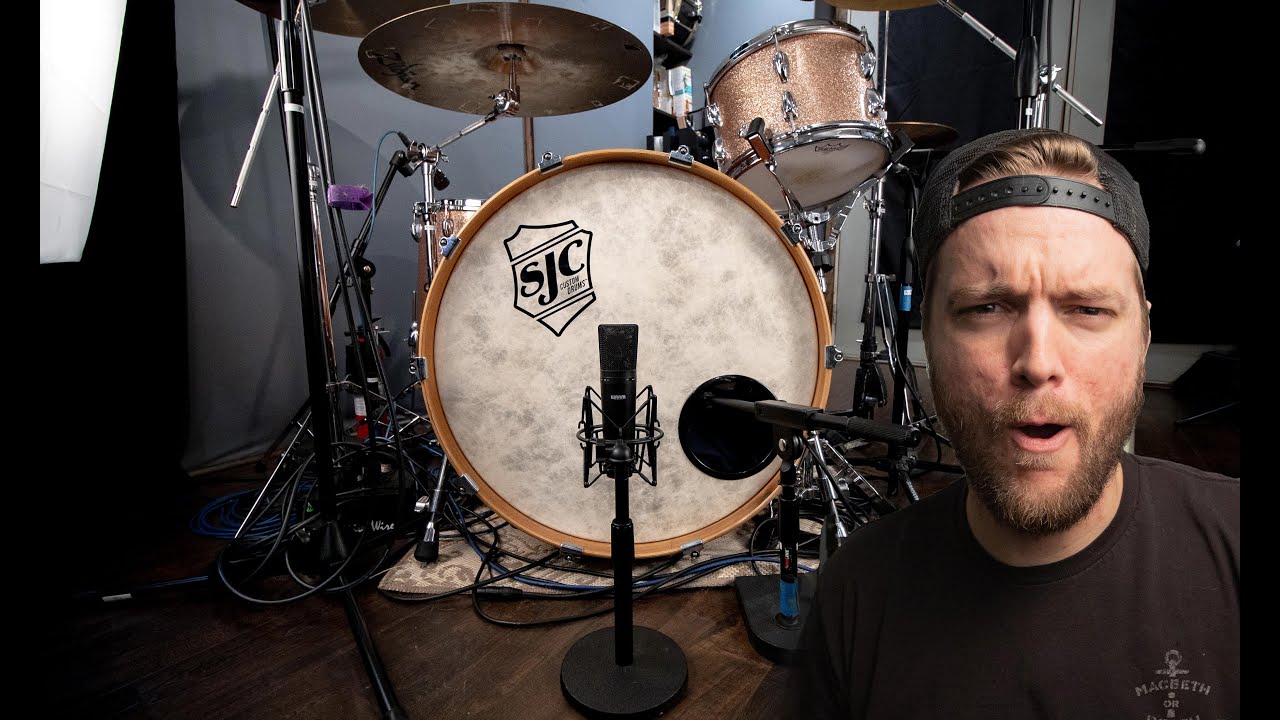The image features a detailed drum set prominently positioned in the center with the focus on the large, white-fronted bass drum that bears a black shield logo with "SJC" inscribed on it. A black microphone is positioned in front of this drum, and another microphone is seemingly placed inside it. Surrounding the bass drum are various bronze cymbals and a smaller tom-tom drum to the right, accented in a goldish bronze hue. The setup is framed by a dark hardwood floor and a light blue wall in the background. 

In the lower right corner of the photograph, a Caucasian man is visible from the chest up. He sports a black t-shirt featuring the "Megadeth" logo on the lower right, although one description mistakenly refers to an anchor and "Macbeth" logo. He has a thin brown mustache and beard, and his backward-facing black snapback hat reveals his blondish-brown hair. The man is facing the camera, squinting his eyes and opening his mouth as if saying "Oh." To the far left, a partially obscured black object, possibly a speaker, with white markings can be seen. The photograph is taken in a landscape layout, accentuating the horizontal expanse of the scene.